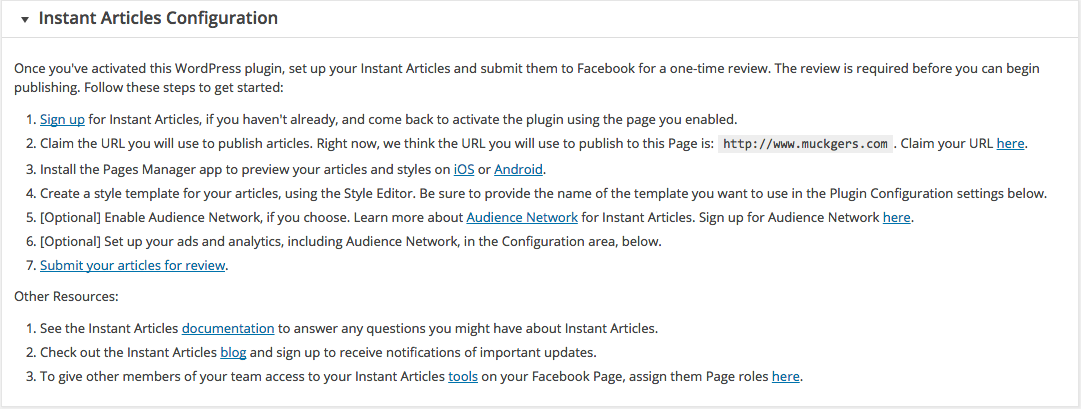Here's the cleaned-up and detailed caption for the image:

---

In the upper left corner, black text reads "Instant Articles Configuration," with a small downward-pointing arrow next to it. Below, the instructions begin: "Once you've activated this WordPress plugin, set up your Instant Articles and submit them to Facebook for a one-time review. The review is required before you can begin publishing. Follow these steps to get started."

1. **Sign Up for Instant Articles** (in blue, underlined text)
2. **Claim the URL** (URL is capitalized; towards the end of the line, "claim your URL here" is underlined in blue)
3. Install the Pages Manager
4. Create a Style Template
5. *(Optional)* Enable Audience Network
6. *(Optional)* Set Up Your Ads and Analytics
7. **Submit Your Articles for Review** (in blue, underlined text)

Next, there's a section titled "Other Resources:"

1. See the **Instant Articles Documentation** (underlined in blue)
2. Check out the **Instant Articles Blog** (underlined in blue)

---